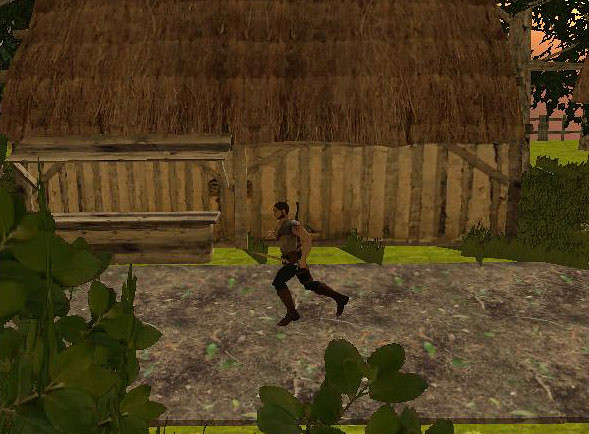In this detailed still image from a video game, a Caucasian male protagonist with short brown hair and a matching short brown beard is captured mid-run at the center of the frame. He is wearing a short-sleeved tan shirt, black pants, and knee-high brown boots, while brandishing a long, pointed sword in his left hand. The background features a rustic, large thatched-roof house constructed from rough-hewn mud and vertical tree trunks. The ground beneath the man appears to be a mix of light and dark gray dirt, adding to the rugged setting. In the lower left corner of the image, rounded green leaves with somewhat pointed tips are visible in the foreground, contributing a touch of vibrant color to the scene.